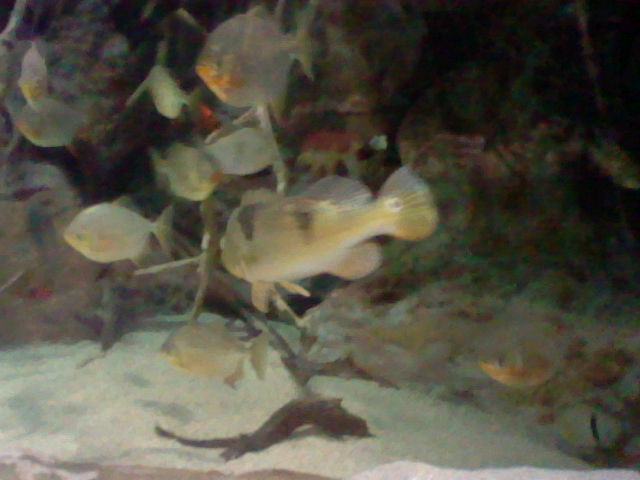This image captures a group of fish swimming in a fish tank. The quality of the photograph is poor and grainy, making the details somewhat unclear and causing the fish to appear slightly out of focus. Despite this, it can be discerned that the tank houses around ten fish of varying sizes. Dominating the scene is a goldish-colored fish with black stripes on its back, positioned front and center. Other fish in the tank display a range of colors including brownish-yellow, off-white, and yellowish hues, some of which exhibit a shimmering effect.

The background of the tank is dark, but various elements are visible, including green leaves, twigs, and underwater branches, suggesting an attempt to recreate a natural habitat. Sand covers the bottom of the tank, along with rock-like structures contributing to the aquatic setting. One particular fish, possibly a sunfish, shows distinct orange coloring on its mouth and belly and swims near the top of the tank. Another notable fish, seen in the middle but not fully visible, appears green with a white belly and distinctive white markings on its top side. The fish are swimming in different directions, adding a dynamic sense of movement to the otherwise blurry and indistinct scene.